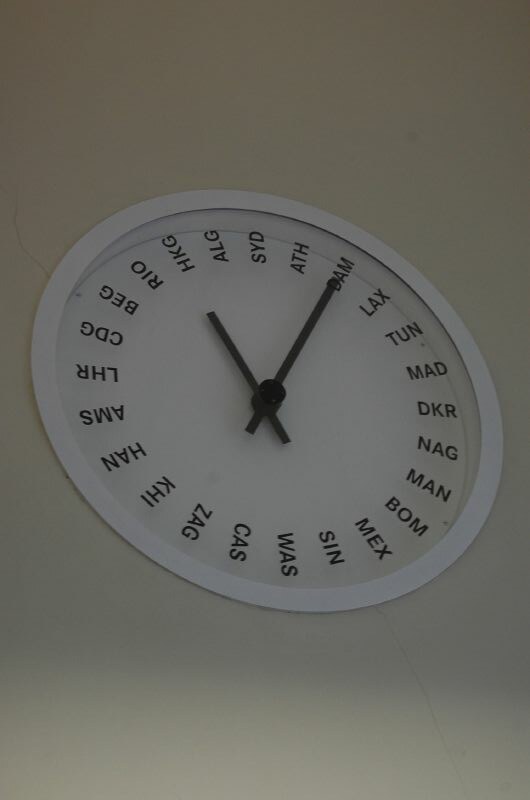A striking, close-up image of a unique wall clock seamlessly integrated into a pristine white wall, featuring a flush white frame that appears as an extension of the surrounding structure. Unlike traditional clocks, this timepiece replaces numbers with an array of three-letter airport codes from cities around the world. Starting from the top and moving clockwise, the codes read: LGA, SYD, ATH, BAM, LAX, TUN, MAD, DKR, NAG, MAIN, BOM, MEX, SIN, WACS, ZAG, KHI, HAN, AMSL, HR, CDG, BEG, RIO, and HKG. Notably, from KHI onwards, the codes appear upside down, creating a visually intriguing element. The current time shows the small hand pointing towards the overlap between HKJ and DAM. The photograph captures the clock from a slightly lower angle on the left side, emphasizing the clock's minimalist design and the spatial interplay between its unique face and the wall.